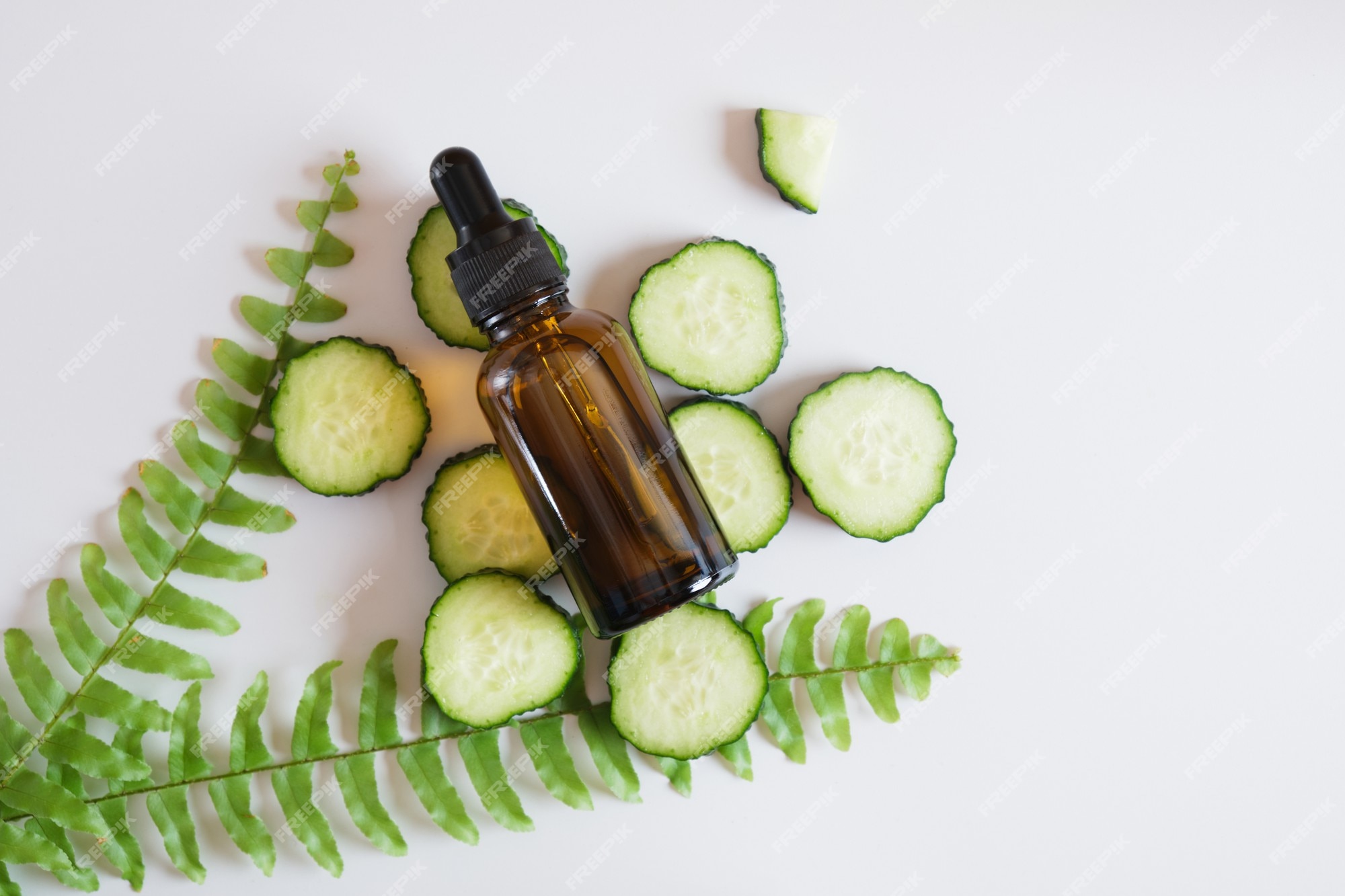The image features a brown, clear glass eyedropper bottle with a black rubber top, stationed prominently on a pile of cucumber slices with dark green skin and pale green insides. These cucumber slices, roughly ten in number, are irregularly spread out, some overlapping others, and occupy the central portion of the image. To the lower left and partially below the cucumbers, two light green fern branches extend diagonally upwards. The background is entirely white, overlaid with a faint, repetitive watermark reading "F-R-E-E-P-I-K" that runs diagonally across the image, making it subtly visible.